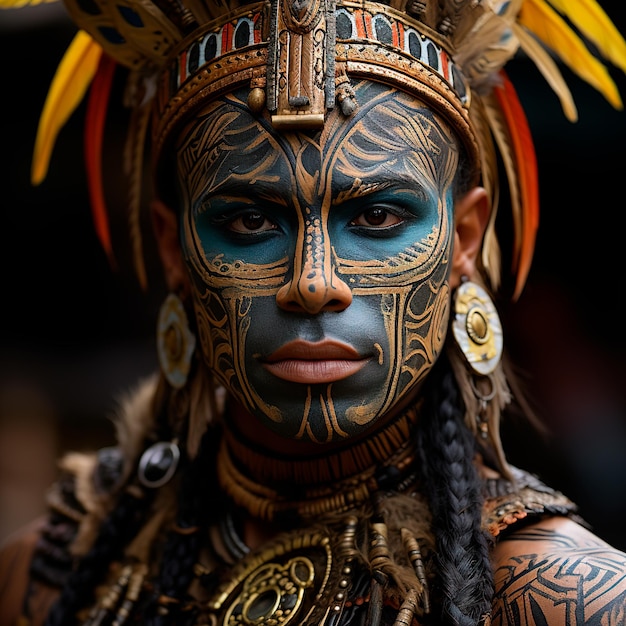The image showcases a high-quality photograph of an individual standing against a black background, emphasizing their intricate appearance. The person is adorned with a tribal headdress featuring yellow, red, and orange feathers, along with leaves. Their face and body are elaborately decorated with ceremonial paint, predominantly green and black, concentrating around the eyes and mouth but extending across their entire face and visible body parts. They have large round earrings in each ear, and their long hair is styled into black braids that drape over their shoulders, with some red hair visible over the left shoulder. The individual's neck is heavily adorned with multiple ornate necklaces, creating a striking layered effect. They sport tribally tattooed arms, adding to the detailed cultural aesthetics. Despite their facial features being fully painted, their focused, unsmiling expression is clearly visible, giving a sense of solemnity and presence. The person’s attire complements the tribal theme, matching the overall ceremonial adornments and tattoos.